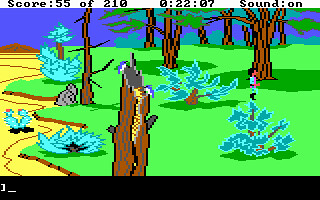This screenshot captures a moment from a pixel art video game, evident from the HUD displayed at the top of the image. The top section of the screenshot features a white bar containing essential game information: "Score: 55 of 210," indicating the player's progress, accompanied by a time stamp reading "0:22:07," and a notation that the sound is turned on.

Beneath this HUD, the main scene depicts a green field in pixel art style. Five trees populate the landscape; notably, two of the trees are dead, with one dead tree prominently in the foreground. Perched on this dead tree is a small pixelated woodpecker, adding a touch of wildlife to the scene. In front of the trees, there are four small bushes colored a light spruce green, which contrast with the deeper green of the field.

To the right side of the image, a hint of a desert biome begins to emerge, suggesting a diverse ecosystem within the game. The bottom edge of the screenshot is marked by a black bar, possibly part of the game interface or a border framing the captured scene.